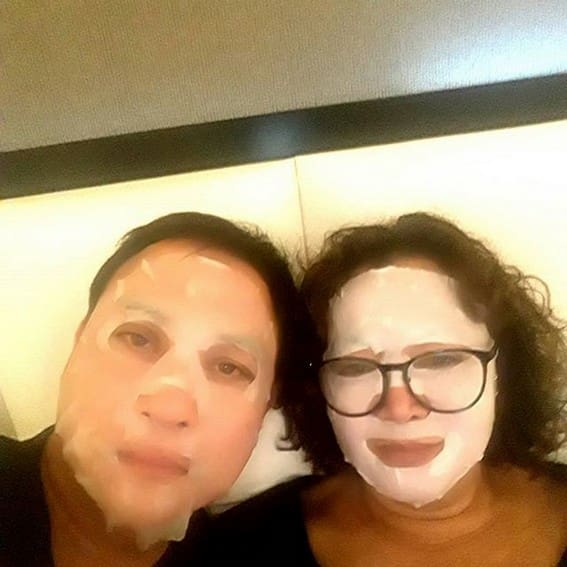The photograph features a man and a woman seated closely together, possibly undergoing a skin care or spa treatment with face masks applied. Both individuals are Caucasian with short brown hair and are wearing black shirts. The man, sitting on the right, has his head tilted towards the woman and is wearing a full white face mask, lending a somewhat sad expression to his face. He also wears glasses with large, brown-rimmed frames. The woman, to the left of him from our perspective, sports a more transparent mask that allows her eyebrows to be visible. Both subjects are not smiling and appear rather serious. They are seated on cushioned seating with a distinct black stripe visible, against a backdrop that includes a grey wall and what seems to be a brown headboard or possibly fluorescent lighting above. The overall image quality is low.